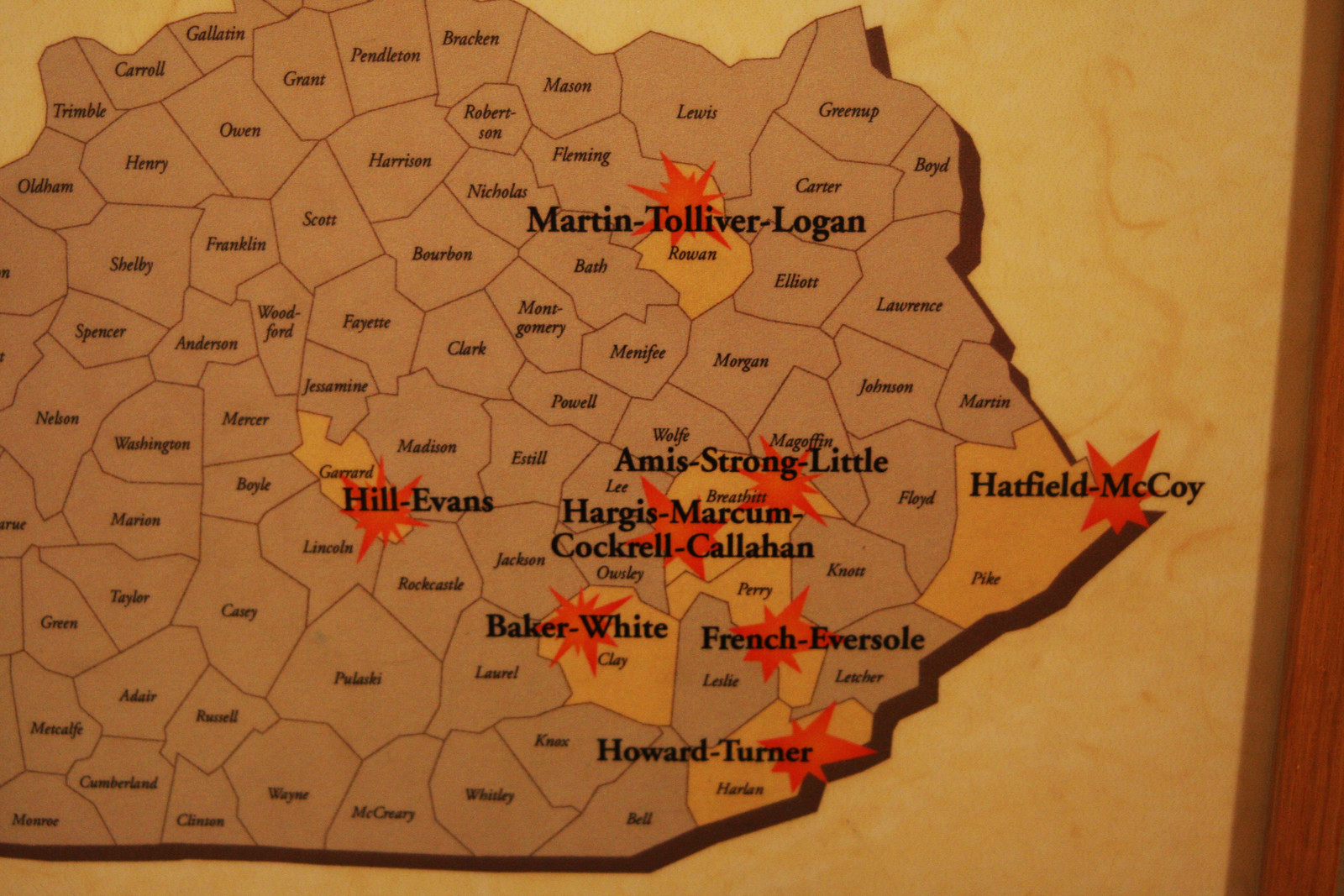The image depicts a detailed map of various counties within a likely state, potentially North Carolina, set against a light yellow, almost cream-colored background with faint, paper-like lines. The map itself is enclosed in a brown wooden frame and appears to be affixed on or crafted into a wall. Each county is outlined and labeled, with the majority of the text rendered in a brown italic serif font for general labels, while notable locations are marked in bold, uppercase serif font and distinguished by an explosive orange star symbol. Counties such as Pike, Harlan, Leslie, Rowan, and others are highlighted with these yellow land areas and orange stars, indicating historical feuds or significant events. Notable labels include "Hatfield-McCoy" in Pike County, "Howard-Turner" in Harlan County, "French-Eversole" in Leslie County, "Baker-White" in Clay County, as well as other feud names like Hill-Evans, Martin-Toliver-Logan, Emmis-Strong-Little, Hargis-Markham-Cockrell-Callahan. Additional counties such as Lewis, Mason, Greenup, Robertson, Harrison, Franklin, Shelby, Spencer, Washington, and Marion are also outlined, albeit in more subdued font styles without the star symbols.